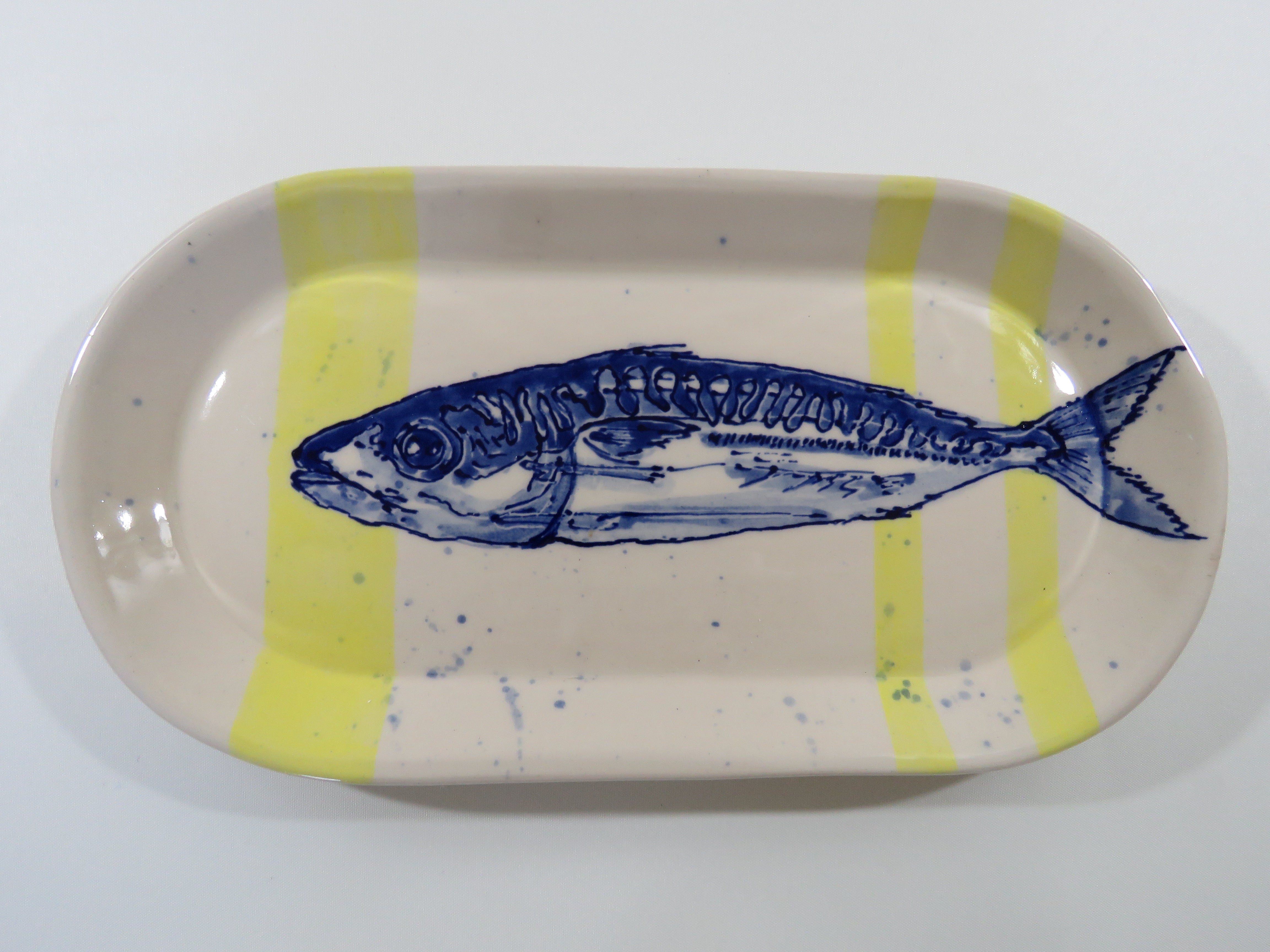This image depicts an oval-shaped dish, possibly ceramic or glass, with a shiny, slightly raised surface more akin to a tray than a plate, set against an entirely white background. The dish, itself white, features a striking design comprising three yellow stripes and blue speckles scattered across its surface. One broad yellow stripe crosses the middle of the dish, while two thinner yellow bands appear on the right side. Over these vibrant accents is a detailed sketch of a blue fish in various shades, including darker and lighter hues. The fish, which appears thin and slightly scraggly, is positioned with its mouth towards the left and its tail fin reaching the right edge of the dish. It has a closed mouth, a split tail fin, and white spots dotting its blue body. The fish’s eye is notably wide open. The arrangement of the stripes places one across the fish's mouth and another across its tail, with the third near its abdomen. Additionally, blue speckles are interspersed throughout, contributing to the visually intricate design. A subtle shadow is cast on both the left and right sides of the dish, enhancing the depth and dimension in the image.